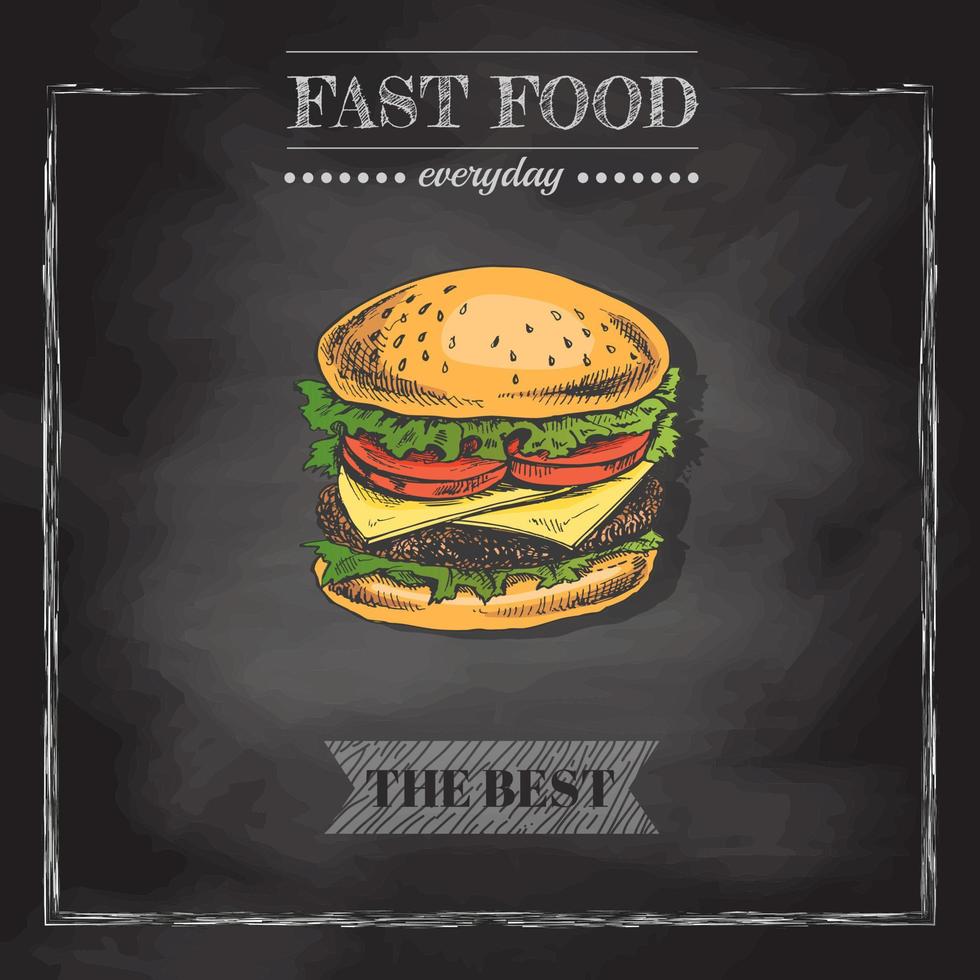The image showcases a restaurant-style poster with a dark black background designed to resemble a chalkboard, complete with chalk remnants and a white inner frame. At the top of the poster, the words "FAST FOOD" are prominently written in a hand-drawn, chalk-like font. Below it, "every day" appears, flanked by small white dots. Centered on the poster is a colorful, detailed drawing of a hamburger featuring a sesame seed bun, two slices of cheese, two tomato slices, layers of lettuce, and a juicy burger patty. At the bottom, within a gray, zebra-like patterned area, the slogan "THE BEST" is boldly displayed, reinforcing the quality of the depicted fast food.